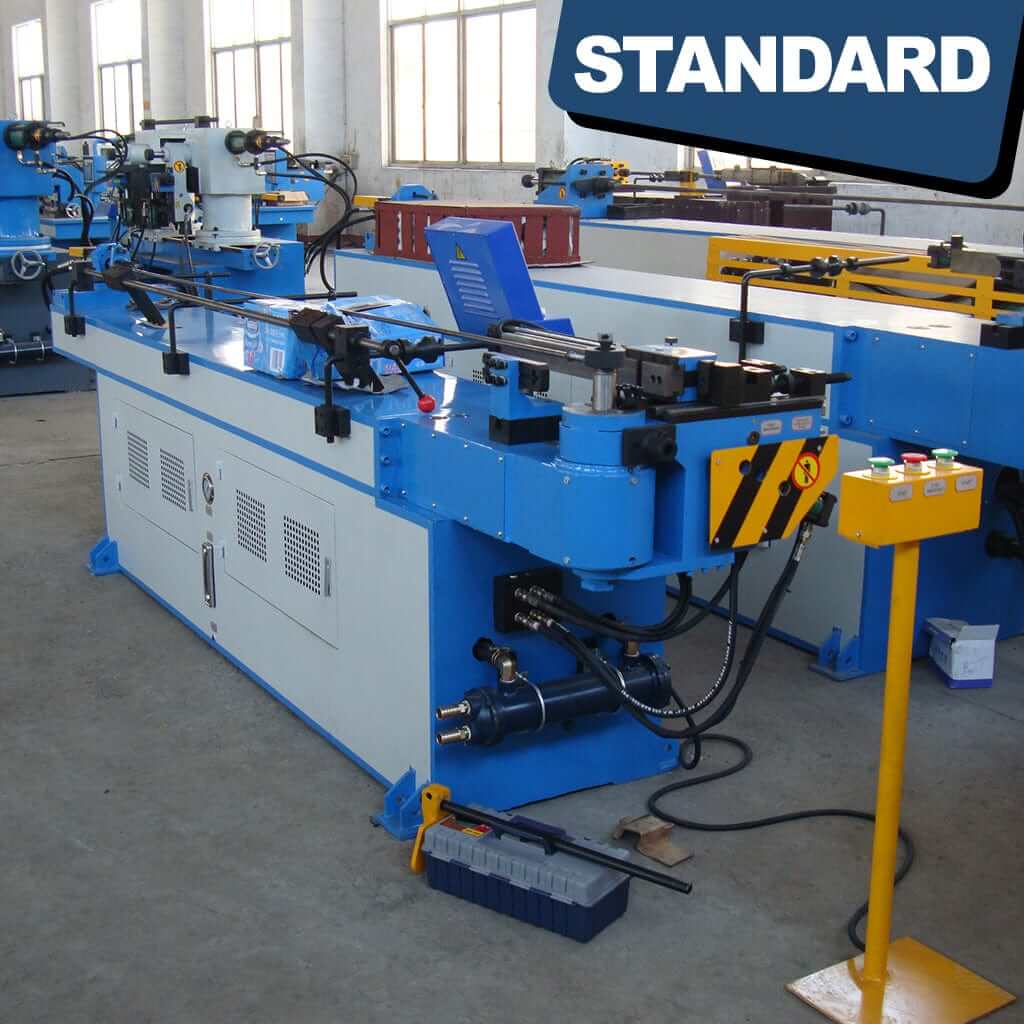This photograph depicts a factory or industrial workshop filled with various large machines, prominently colored in blue, gray, and yellow with black caution stripes. In the top left corner, white text on a blue background reads "standard." The center of attention is on a significant piece of machinery that appears akin to a table with metal bars and what might be an industrial lathe, with various knobs suggesting cutting functions. This blue machine has black metal rods running across it, contributing to its intricate appearance.

To the side, there's a yellow control panel featuring diagonal black stripes, emitting a sense of industrial caution. Several black cords connect the blue machinery to another yellow structure, which consists of a square base supporting a cylindrical pole. This structure is topped with a rectangular yellow box equipped with three buttons: two green and one red, configured for machine operation.

Additionally, there’s a red box located upside down on a ledge nearby and a navy blue and gray toolbox with a yellow accent rests on the floor. The area is well-lit through large windows with whited-out panes, suggesting it’s daytime. The floor of the establishment seems concrete but gives off a carpeted appearance in the photo, adding to the utilitarian ambiance of this industrial setting.